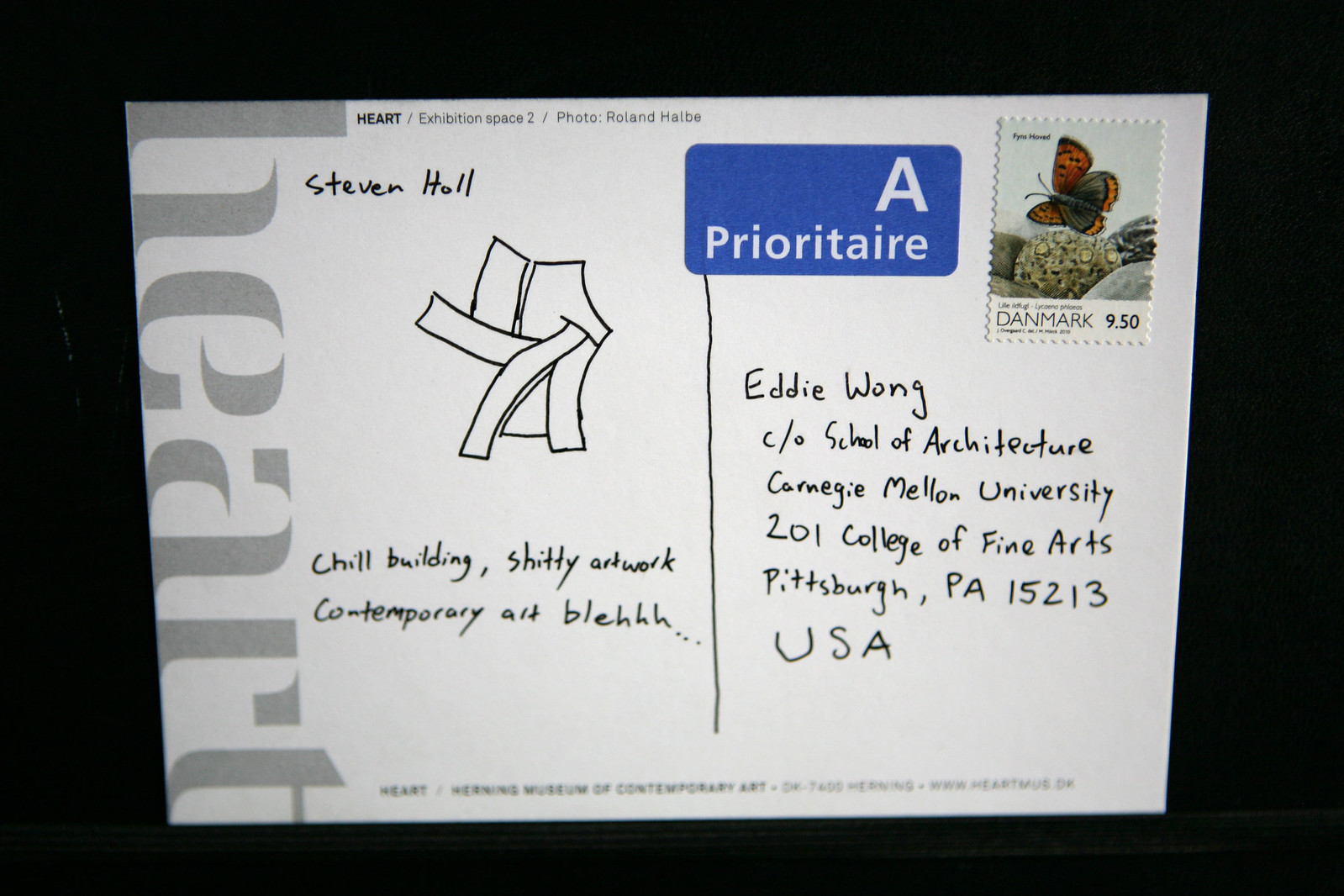The image features a color photograph in landscape orientation with a black background framing a horizontally aligned postcard. On the top right corner of the postcard, there is a stamp depicting a red-orange butterfly with the inscription "Danmark 9.50". Adjacent to the stamp is a dark blue sticker with a large white capital letter "A" and the word "Prioritaire" beneath it in white text.

The postcard is addressed to Eddie Wong of the School of Architecture at Carnegie Mellon University, 201 College of Fine Arts, Pittsburgh, PA, 15213, USA. This address is written in black ink and handwriting. On the left side of the postcard, there is a name, Stephen Hall, printed in a non-cursive font, accompanied by an abstract line art illustration. Below the illustration, the text "Chill Building, Shitty Artwork, Contemporary Art, Blehh…" is written in handwriting. 

Additionally, along the left margin of the postcard, there is vertical gray typography that spells out "HEART" in large lowercase letters. The juxtaposition of the intricate stamp, detailed address, and the expressive text and illustration adds a layer of depth to the postcard, blending formal and casual elements in a distinctive, personalized manner.